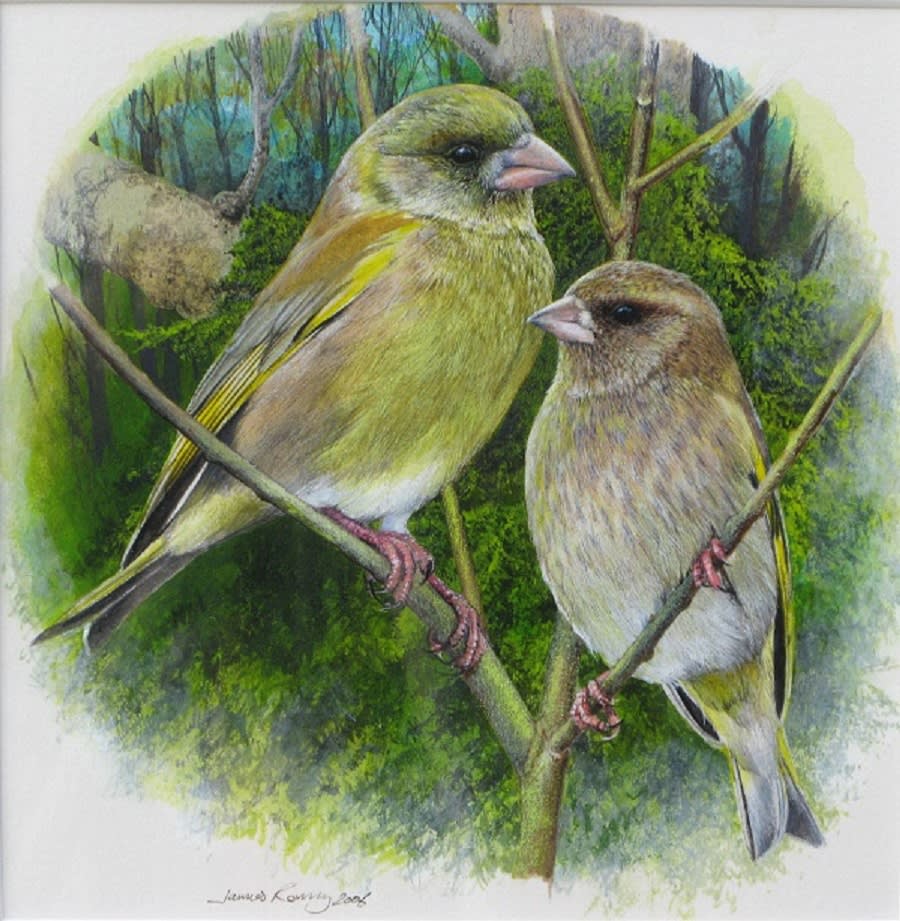This image displays a detailed painting of two birds perched on a branch amidst a lush, forested background, characterized by verdant greens, earthy browns, and hints of blue. The two birds, likely representing a male and a female, are positioned with one bird slightly higher and looking to the right, and the other bird a bit lower and glancing to the left. The birds, predominantly yellow with notable orange beaks and some black markings along their tails, seem to gaze past one another, creating a subtle dynamic in their poses. The painting is uniquely rendered within a circular frame, leaving the four corners of the square canvas untouched and white. The artwork is signed "James Rory, 2006" at the bottom, adding an authentic personal touch to this vibrant and textured depiction of nature.